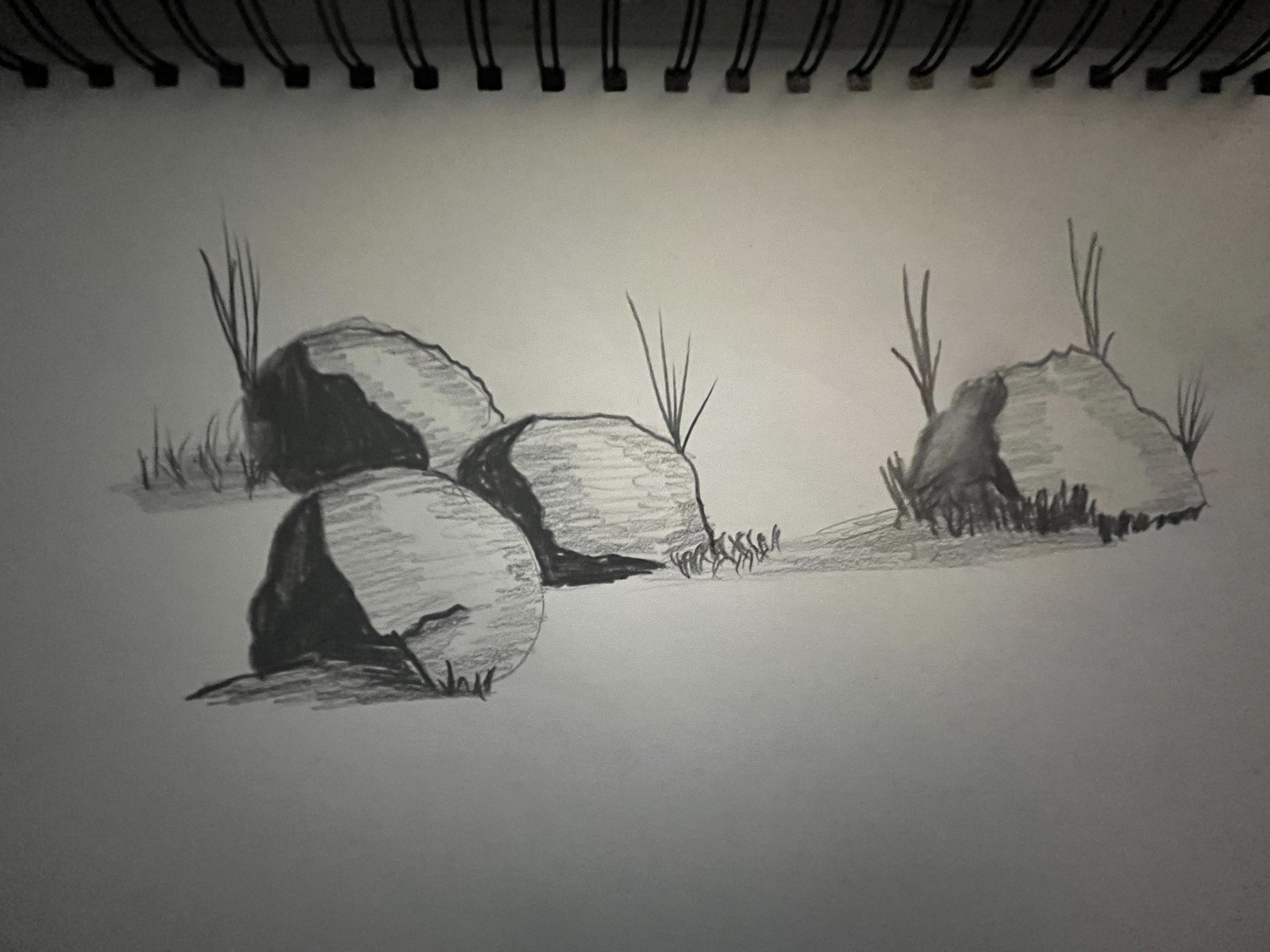In this horizontally elongated rectangular image, a sketch pad, typically used by artists, is prominently featured with its spiral binder aligned along the top edge of the photo. The open page of the sketch pad showcases an intricate drawing of four large, weathered boulder rocks. Each boulder is meticulously shaded, with the light source illuminating the right side of the rocks, creating stark, darkened shadows on their left sides. Behind the rear three boulders, tufts of long grass are depicted, adding depth to the scene. In contrast, short grass patches are sketched around the base of these rocks. As the viewer's eye travels downward on the illustration, the paper's tone transitions into a shadowy, darkened hue, enhancing the overall atmospheric effect of the drawing.